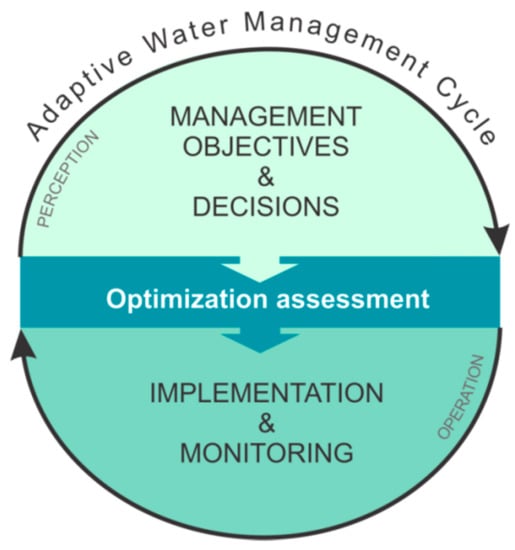The image displays an infographic titled "Adaptive Water Management Cycle" set against a white background. It features a circular flow depicted by a series of black arrows. The top semi-circle is filled with a light green color, the middle horizontal stripe is blue, and the bottom semi-circle is darker green. The text within the light green area at the top reads "Management Objectives and Decisions" in black, and it includes the word "Perception" in gray on the left. The middle blue section, marked by white text, reads "Optimization Assessment" with two arrows moving through it, indicating the transition between the top and bottom sections. The bottom darker green area, with "Implementation and Monitoring" in black, also features the word "Operation" in gray. This visual representation demonstrates the continuous cycle of perception and management objectives leading to optimization assessment, which then progresses to implementation, monitoring, and operation, illustrating a systematic approach to adaptive water management.